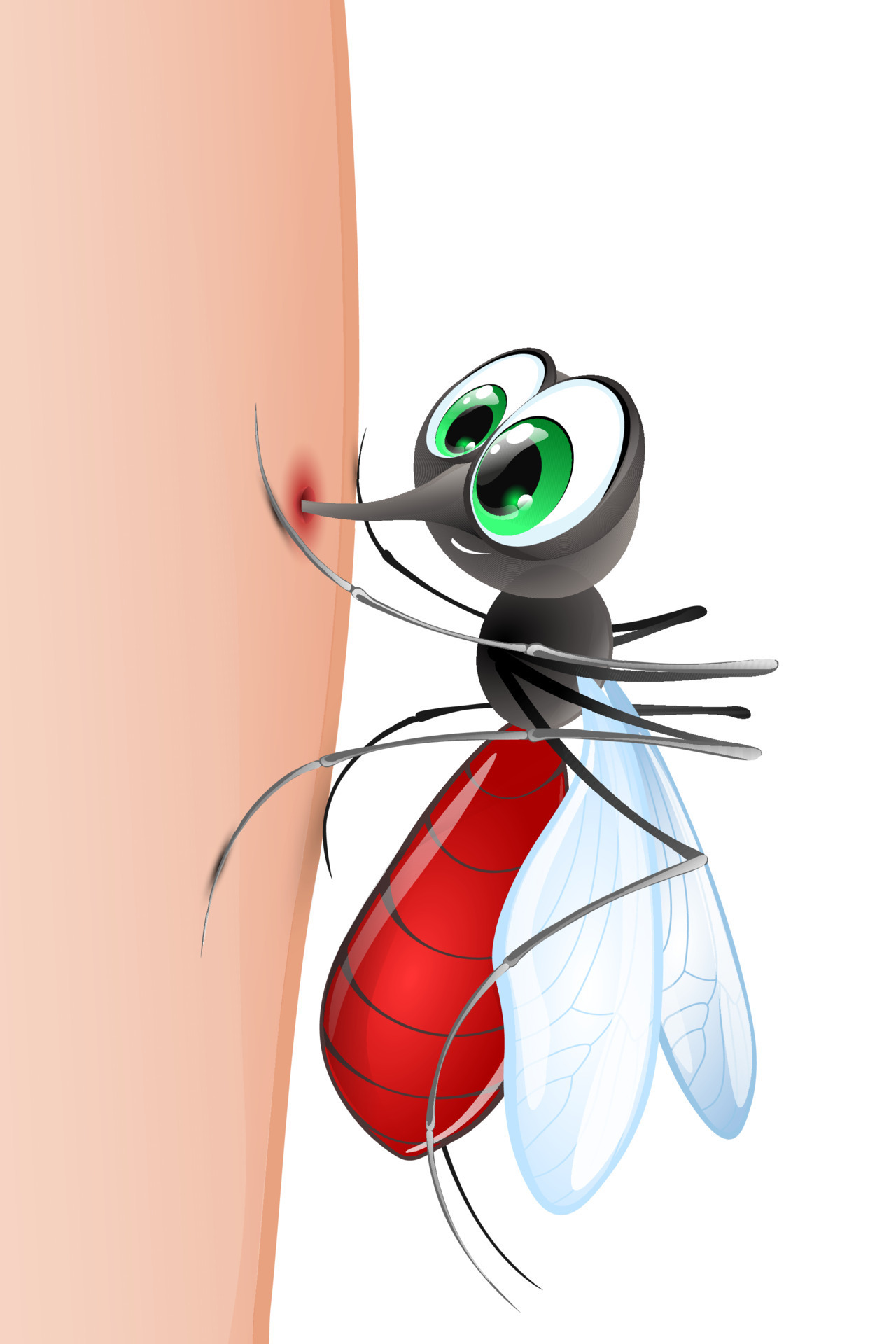In this whimsical and animated drawing, a comical, oversized mosquito is depicted biting into a person's arm, shown as a large, tan-colored expanse with a prominent red dot marking the sting site. The mosquito, rendered in a cute and playful cartoon style, has an almost cheerful expression despite the potentially "scary" scenario. Its head and upper body are black, while its abdomen is distinctly red, suggesting it’s filled with blood. The insect’s large, bright green eyes are outlined in white, adding to its exaggerated, endearing look, and its tiny, smiling mouth even reveals some teeth. Its translucent white wings and six legs are meticulously drawn, highlighting the mosquito’s exaggerated size compared to the arm. The overall image, set against a whitish background, combines elements of pain and humor, making the mosquito appear both threatening and amusing.